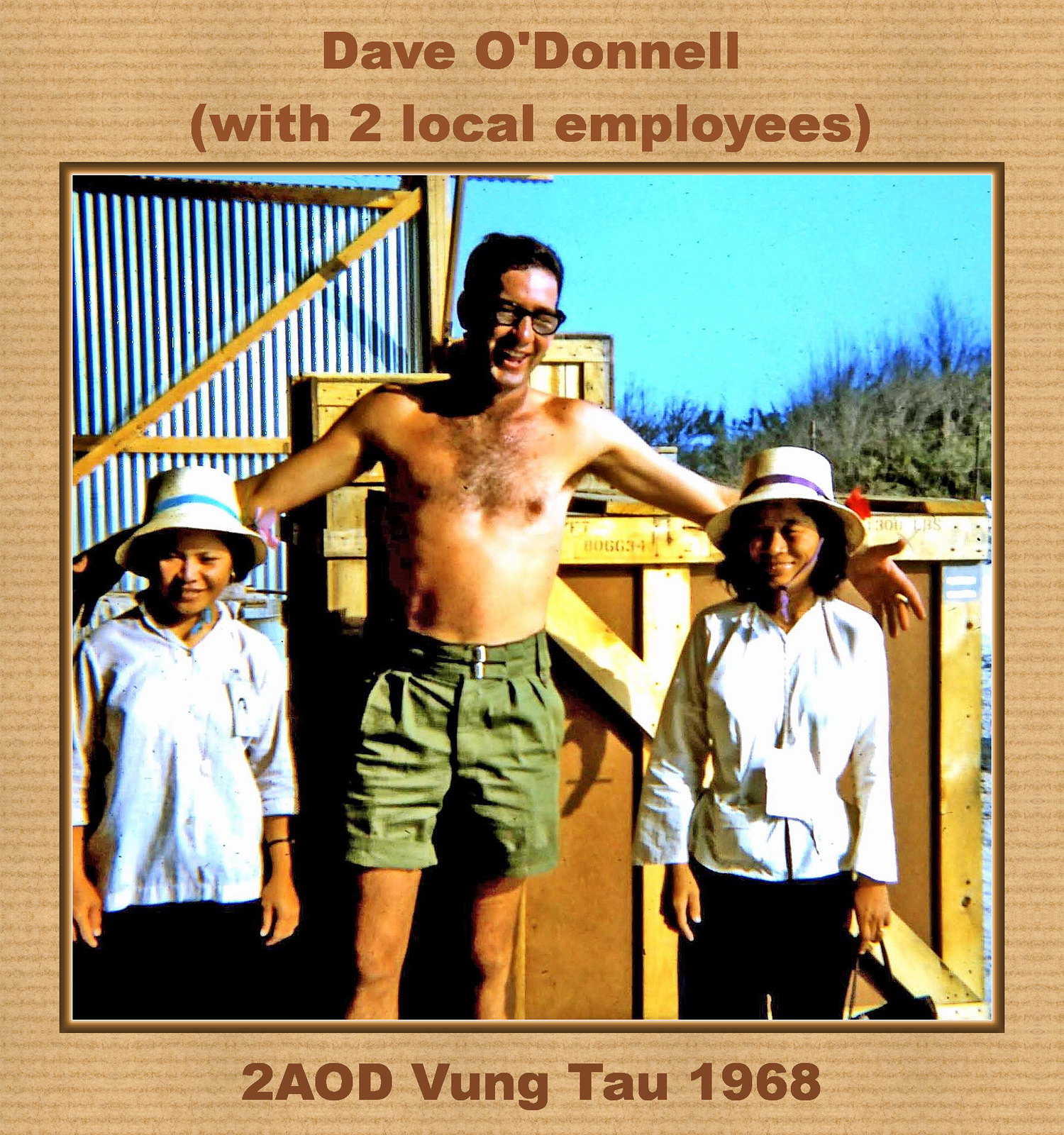This square, framed photograph from 1968, bordered by sturdy brown cardboard, captures a striking scene in Vung Tau. Central to the image stands a very tall, shirtless Caucasian man, identified by the brown text at the top border as "Dave O'Donnell (with two local employees)." His attire includes army-green dress shorts, and he sports short black hair and black-rimmed glasses. His arms are stretched out behind two petite Asian women, appearing as though he's embracing them without actually touching. The women, likely Vietnamese and significantly shorter than Dave, are positioned to his left and right, each donning Panama-style hats with ribbons—blue for the woman on the left and purple for the woman on the right. They wear matching white shirts and black pants. In the background, trees and some distant boxes provide context to the outdoor setting. The bottom border of the photo is inscribed with "2AOD Vung Tau, 1968."